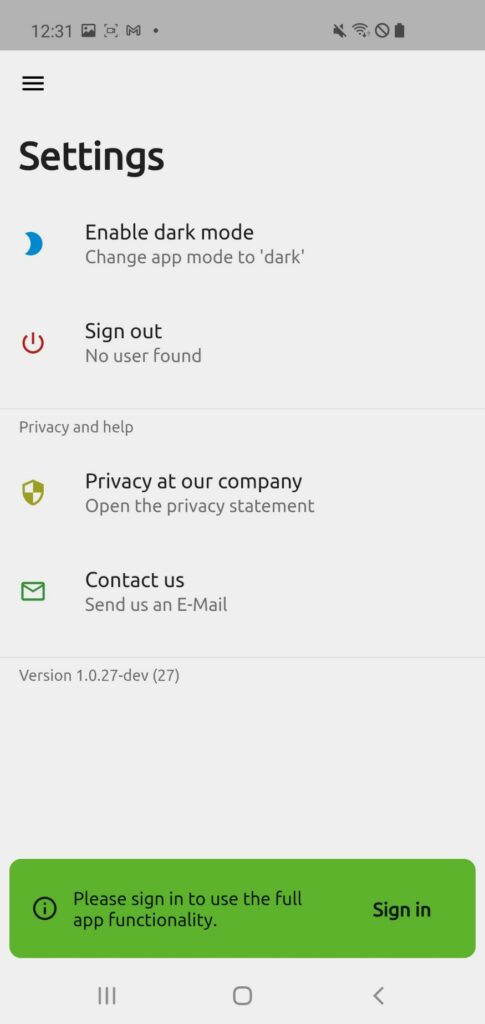In the image, we are presented with the settings screen of a cell phone app. The top left corner displays the time as 12:31, with three cell phone signal icons next to it. Surrounding this area is a gray background. Below, occupying almost the entire screen from top to bottom, is a light gray background featuring the settings menu. 

The menu begins with the heading "Settings" in black letters. Following this, there is an option labeled "Enable Dark Mode." Further down is the "Sign Out" button. Underneath these options, in smaller gray text, are "Privacy and Help." The next item reads "Privacy at our company," followed by "Contact Us" and "Send Us an Email."

Each category has an icon to its left: 
- A blue moon icon for "Settings."
- A red power button for "Sign Out."
- A shield, half white and half brownish-green, for "Privacy at our company."
- A green email icon for "Send Us an Email."

At the very bottom of the screen, there is a message in black text stating, "Please Sign In to Use the Full App Functionality," followed by a "Sign In" button in black text on a green background. Finally, at the extreme bottom of the screen, there are three navigation icons: three vertical lines on the left, a circle in the middle, and an arrow pointing to the left on the right-hand side.